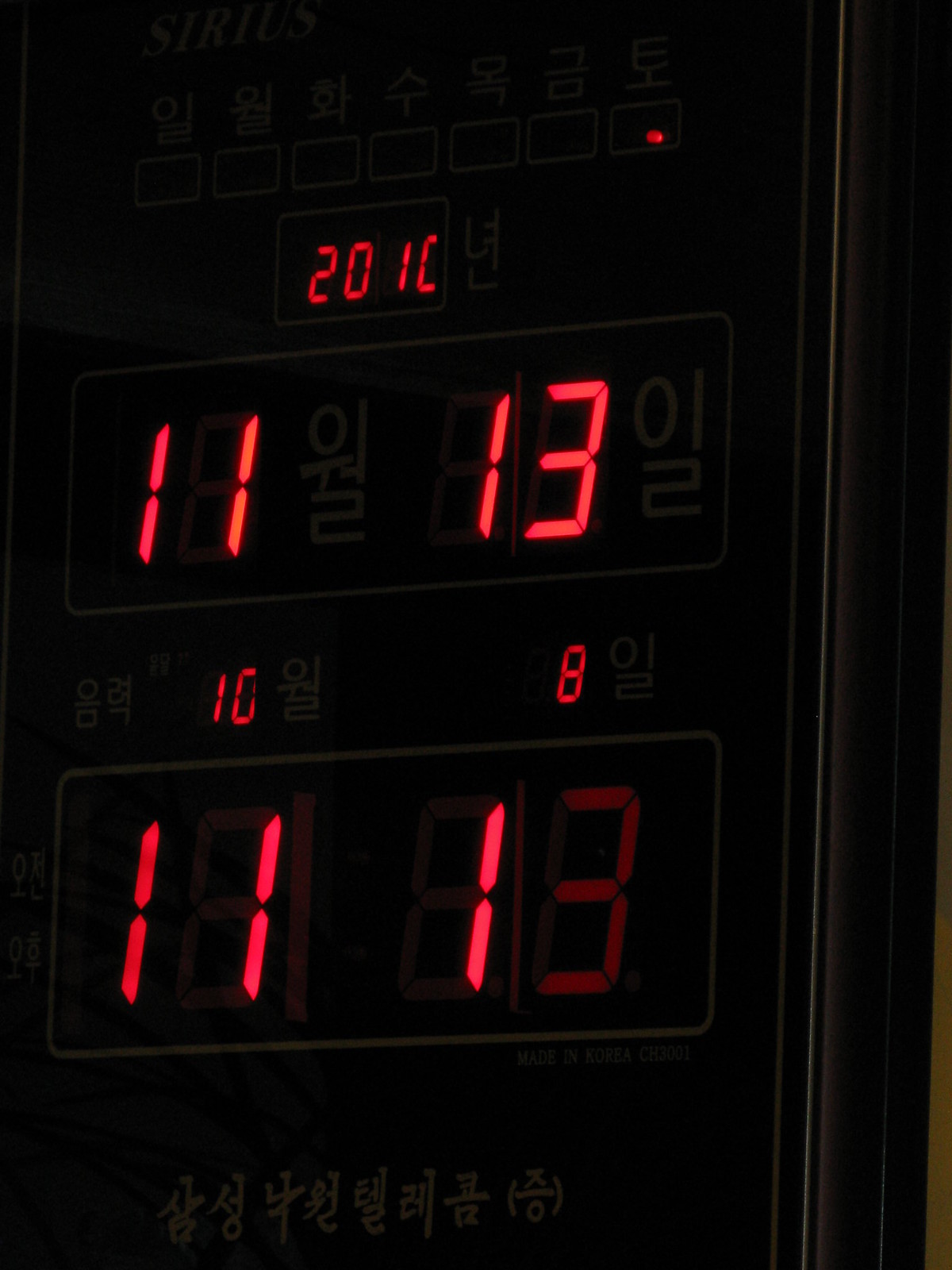The image features a black background with glowing red numbers, reminiscent of an LED display or scoreboard. At the top, "21c" is displayed in red. Below this, on the bottom left, the number "11" is lit in red. On the bottom right, the number "13" is brightly displayed. Beneath these numbers, in a smaller font, "10" and "8" are shown. The very bottom line displays the numbers "11" and "1" in a glowing red, with the "3" appearing slightly dimmer. Additionally, there is some Chinese lettering at the bottom. The overall scene is dark, with the red numbers providing the primary light source, giving it an eerie, illuminated effect.